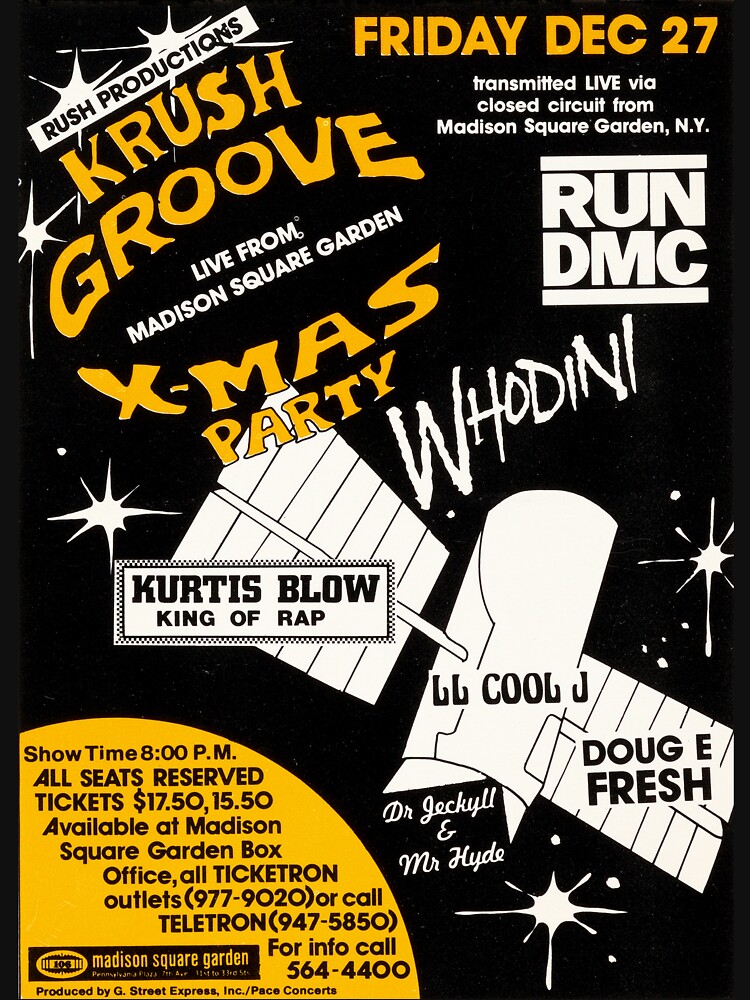This vibrant poster advertises an exclusive Crush Groove Xmas Party, showcasing an ensemble of top hip-hop artists. Set against a stark black background, the text is predominantly white and yellow. In the top right corner, in yellow, the date is highlighted: Friday, December 27th. Just below it, the white text states, “transmitted live via closed circuit from Madison Square Garden, New York.” Prominently positioned at the center, it announces: “Live from Madison Square Garden.” 

Key performers are listed: Run DMC, Houdini, Curtis Blow, King of Rap, LL Cool J, Doug E. Fresh, and Dr. Jekyll and Mr. Hyde. Surrounding these names is a white, satellite-like image, adding a futuristic touch, with drawings of stars scattered across the black sky. To the left, the organiser is identified with “Rush Productions” in bold white text on a contrasting black background.

In the bottom left, a conspicuous yellow half-circle provides essential details: Showtime at 8 PM, ticket prices at $17.50, along with additional information about the venue, tickets available at the Madison Square Garden box office and all Ticketron outlets, and a contact phone number for inquiries (564-4400). The overall design, with the mix of white, yellow, and occasional orange fonts, not only draws attention but effectively communicates the essential details of this exciting event.